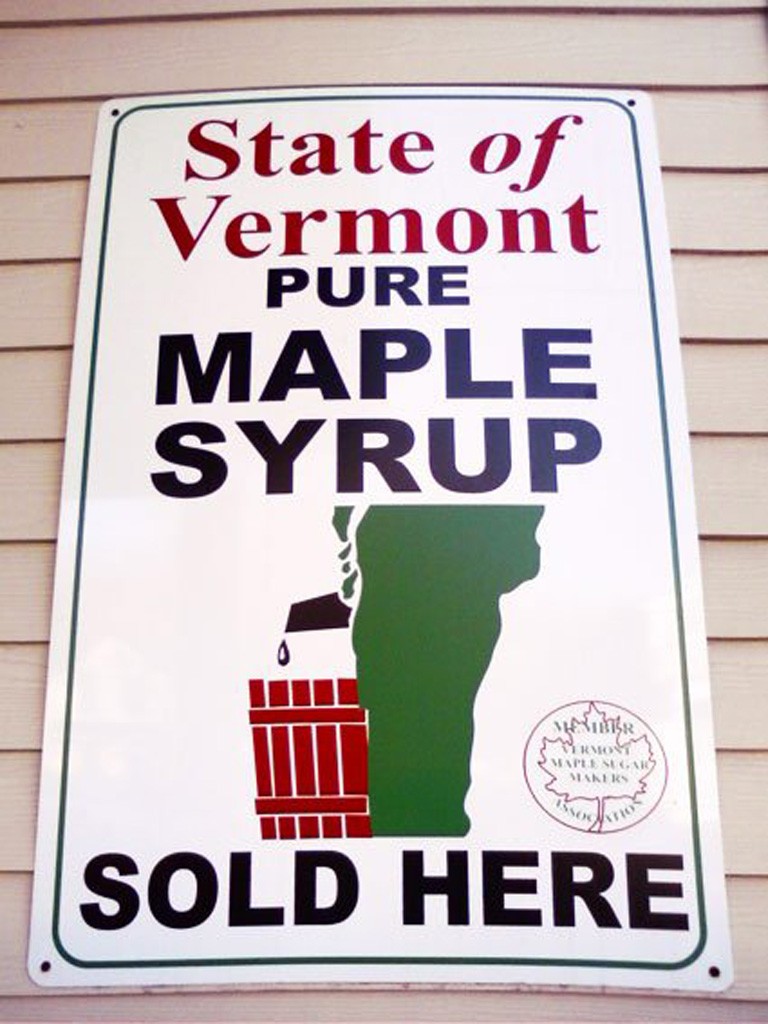Affixed to the side of a house with light pink paneling, almost entirely covering the image, is a vertical, rectangular white sign with vibrant text and graphics. The sign features the following elements:

1. At the top, in bold red letters, it reads "State of Vermont".
2. Directly below, in blue letters, it states "Pure Maple Syrup".
3. Centrally, there is a green silhouette of the state of Vermont.
4. To the left of the Vermont shape and touching it, a red depiction of a five-plank fence appears, potentially symbolizing a bucket.
5. A black faucet extends from the Vermont shape, dripping a liquid into the red fence, creating an unfortunate visual that may be perceived humorously as a man urinating into a bucket.

Beneath this graphic, in black letters, the sign reads "Sold Here". Above the word "Here", there is a circular logo featuring what seems to be a maple leaf. The text around the logo is partially legible, possibly stating "Vermont Maple Sugar Makers Member".